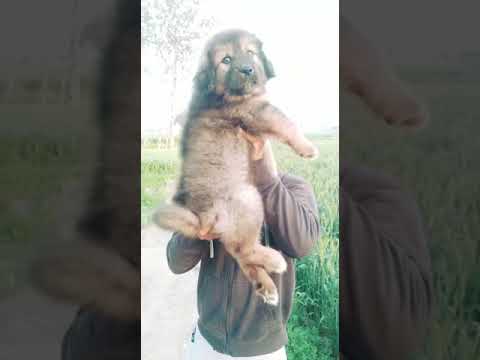In the image, a person is holding a young, furry puppy with floppy ears. The puppy is primarily tan with black and white markings, including a black and tan head and white-tipped feet. The person's face is completely obscured by the puppy. They are dressed in white sweatpants and a grey jacket. Behind them lies a green field of grass with a tree visible at the top left corner of the picture. The individual is standing on a cement sidewalk that traverses the middle of the image. The sky above is grey with no visible sun or clouds, suggesting overcast weather. The scene likely takes place in a park, lending a serene, natural backdrop to this candid and charming moment where the playful puppy steals the spotlight.